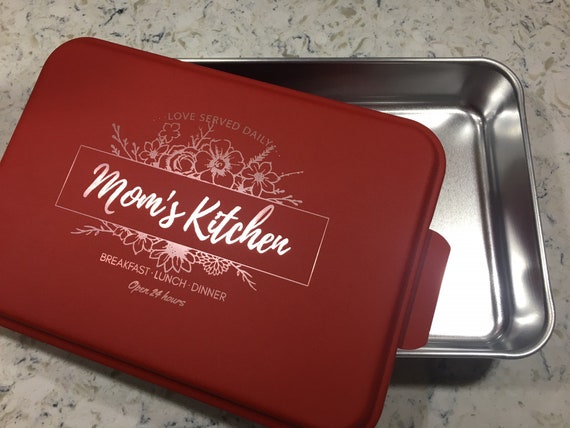The image depicts a rectangular, metal container resembling a lunchbox or baking dish with a snap-on lid. The lid is a burgundy red color and features decorative flower etchings. Prominently centered among the flowers, there is a white rectangular label with the cursive inscription "Mom's Kitchen." Below this, the words "Love Served Daily" are displayed, and further down, it lists "Breakfast, Lunch, Dinner, Open 24 hours." The container is situated on a smooth, white marble countertop, emphasizing its vibrant color and detailed design. The latches attaching the lid to the container are also visible, adding to the overall practicality and charm of the piece.